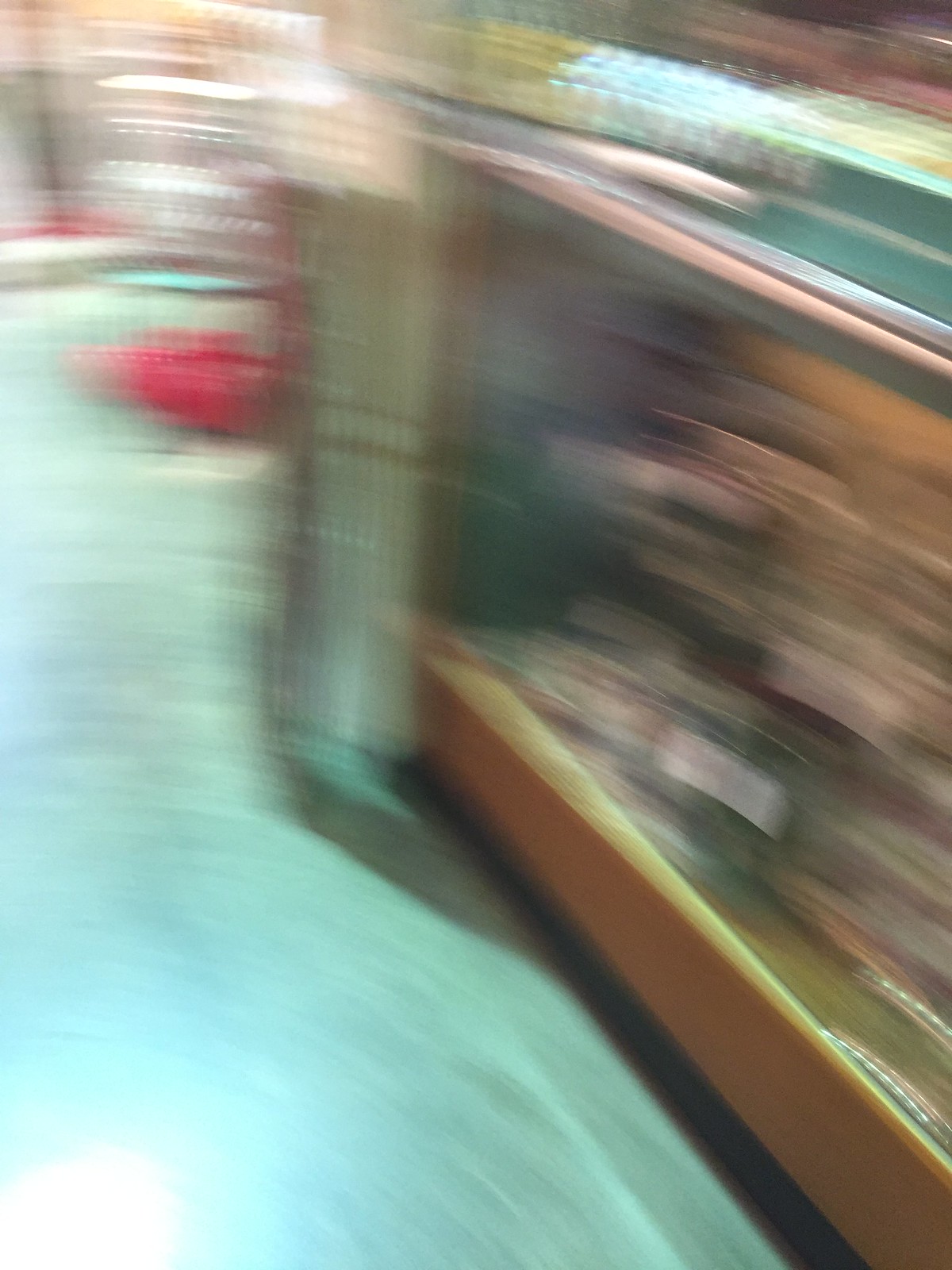This portrait-oriented photograph is heavily blurred, making the details indistinguishable. A diagonal feature, possibly a pathway or a concrete floor, extends from the bottom right to the top left. The bottom left corner is illuminated by a bright light, contrasting with the rest of the image. There appears to be a display case along the right side, but it remains indiscernible due to the blur. Towards the top left on the floor, a red object is visible, though the motion blur suggests rapid movement, potentially indicating someone spinning around. The overall scene is indecipherable, characterized largely by its intense blur and indistinct elements.